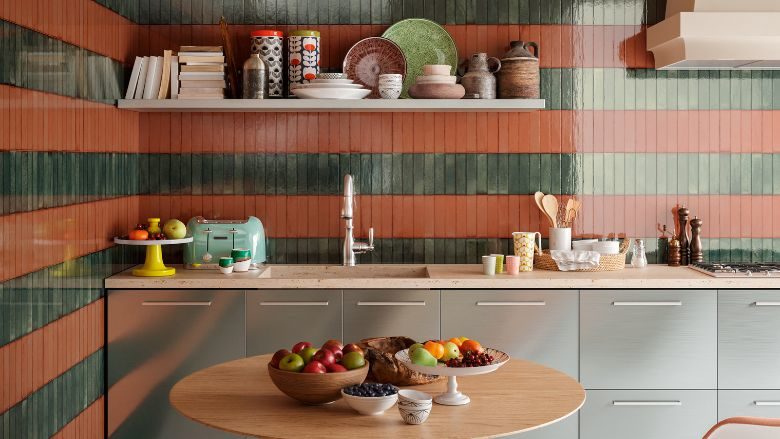The image shows a kitchen with a distinct tiled pattern of alternating rows of brown and green tiles on two perpendicular walls. A prominent feature is the white shelf mounted on the wall directly facing the camera. This shelf is organized into three sections: books are placed on the left, plates and bowls in the center, and various containers — some of which are white with green and red tops — on the right. Below the shelf, a white marbled countertop supports a sink, which has light gray cabinets with thin, flat handles underneath it. To the left of the sink, a yellow stand holds a plate of orange grapes and pears, while to the right, there are several cups. 

In front of the sink, a round wooden table anchors the setting, featuring bowls of fruit. One bowl is filled with red and green apples and another with blueberries. An additional white platter contains a mix of oranges, pears, and cherries, accompanied by two stacked bowls and something that resembles an orange bread-like item.